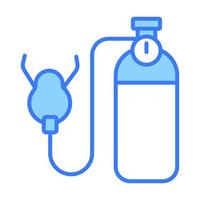This image is a simplistic, cartoonish PNG or vector icon set on a white background, designed in a style reminiscent of an emoji or medical slideshow. It depicts an oxygen mask and tank using very basic lines and minimal detail. The oxygen mask is light blue with dark blue edging, which connects via a blue line that extends to the left and then down to the oxygen tank. The tank itself is divided into a top blue section outlined in blue and featuring a blue-outlined circle containing a white dial with a dark blue center. The bottom part of the tank is white. The overall drawing is devoid of text and has a clean, uncomplicated look, suitable for instructional materials or digital icons.